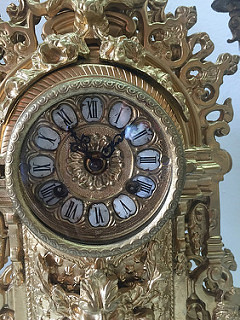This photograph captures a close-up of an ornate, gold-colored clock set against a light blue background. The clock exudes a sense of royalty and antiquity, reminiscent of something that might be found in a regal setting. The clock is intricately designed with elaborate leaf-like patterns and curly designs that culminate in delicate tips. The clock face is adorned with Roman numerals from I to XII, each set against a round, gray backdrop. The clock hands, black and intricately designed, point to 1:55. In the center of the clock face is a circular area that resembles a flower, adding to the clock’s elegantly antique appearance.